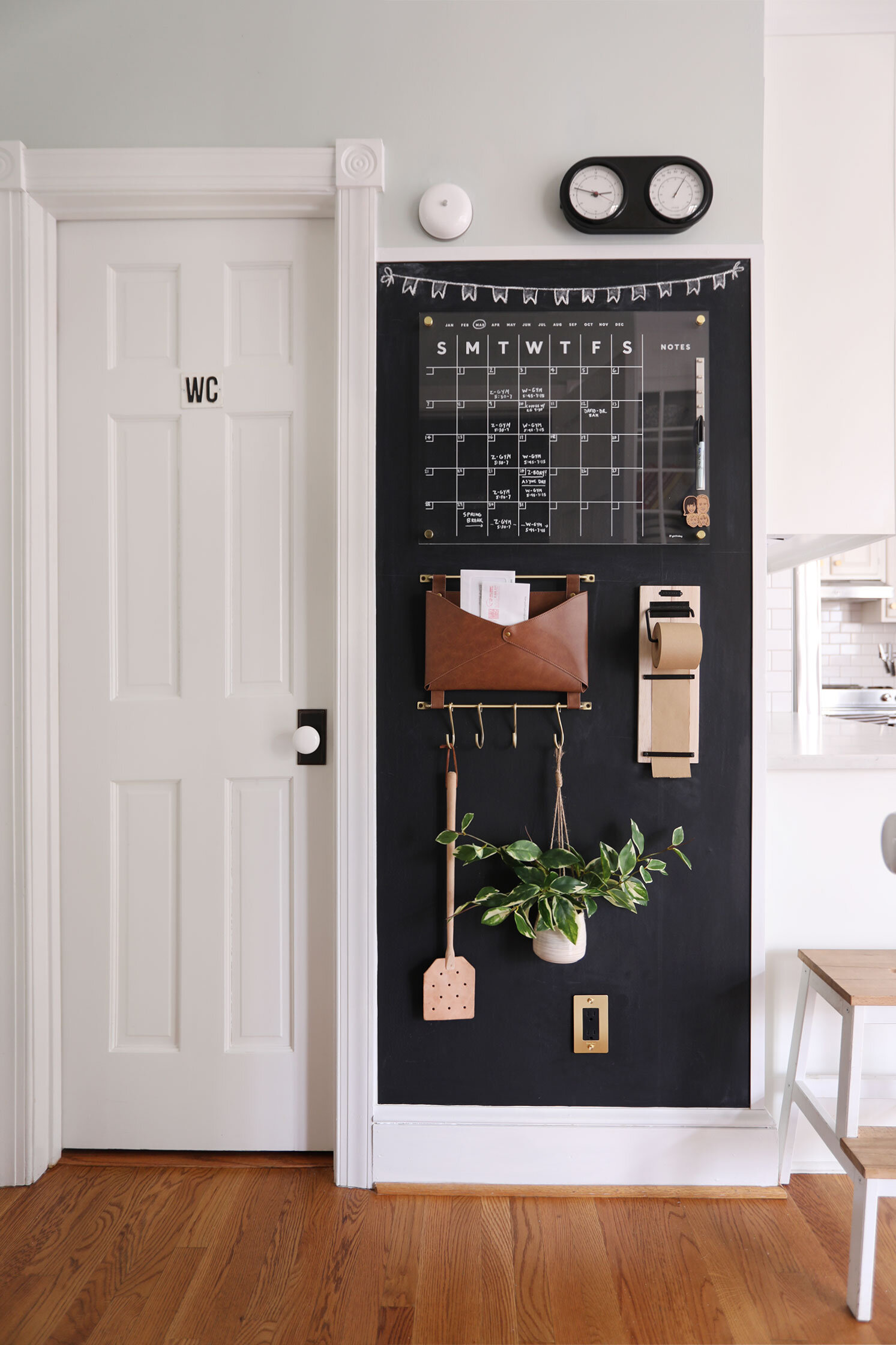The photograph features an indoor scene of what appears to be a kitchen area in a residential house. The floor is made of light brown hardwood slats. On the left side of the image is a closed white door with a matching white frame, labeled "WC" in black capital letters at the top, indicating it is a water closet (bathroom). Next to the door, on the right, is a black section of the wall that seems to be either painted with chalkboard paint or covered with a black material. At the top of this black section, there is a calendar labeled with white capital letters "SMTWTFS" for the days of the week, and each day is divided into uniform squares with dates numbered in the upper left corner. 

Below the calendar, there is a dark brown large envelope affixed to the wall, containing a couple of white envelopes, likely for holding mail. Further down, a fly swatter is suspended from a hook, and there is a green plant in a white pot hanging from another hook. Positioned at the top of this black section is a clock. Additionally, there is mention of a little stool or bench against another white wall to the right, suggesting that the area further to the right leads deeper into the kitchen.